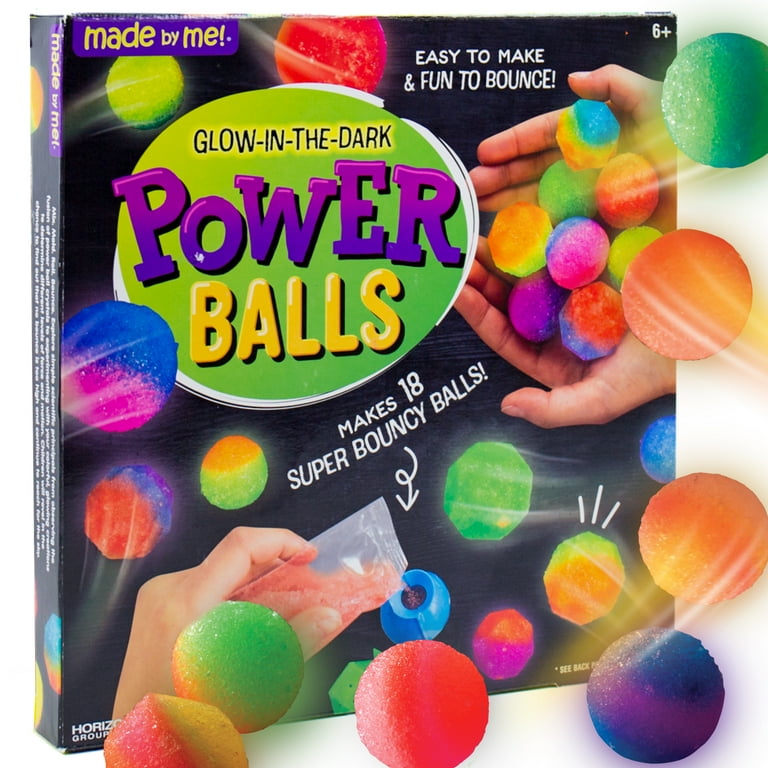This image showcases a vintage-styled, black packaging of a kit used to create glow-in-the-dark power balls, marketed as "easy to make and fun to bounce." The box advertises the ability to make 18 super bouncy balls in a variety of colors. Dominated by bold and playful text, "Glow-in-the-Dark" is in blue, "Power" is in a large, all-caps purple gradient, and "Balls" appears in large yellow letters against a green oval with a white outline. The upper left features "Made by Me" in purple and yellow. The center of the package displays a hand pouring powder into a mold, illustrating the creation process. Additional images show a variety of multicolored balls including red, blue, green, purple, orange, and pink, with some hands cradling a collection of them. These balls vary in shapes and sizes, some perfectly round, others resembling geometric dice-like forms. The packaging and the dynamic presentation of the product emphasize the playful and engaging nature of creating these vibrant, bouncy balls.